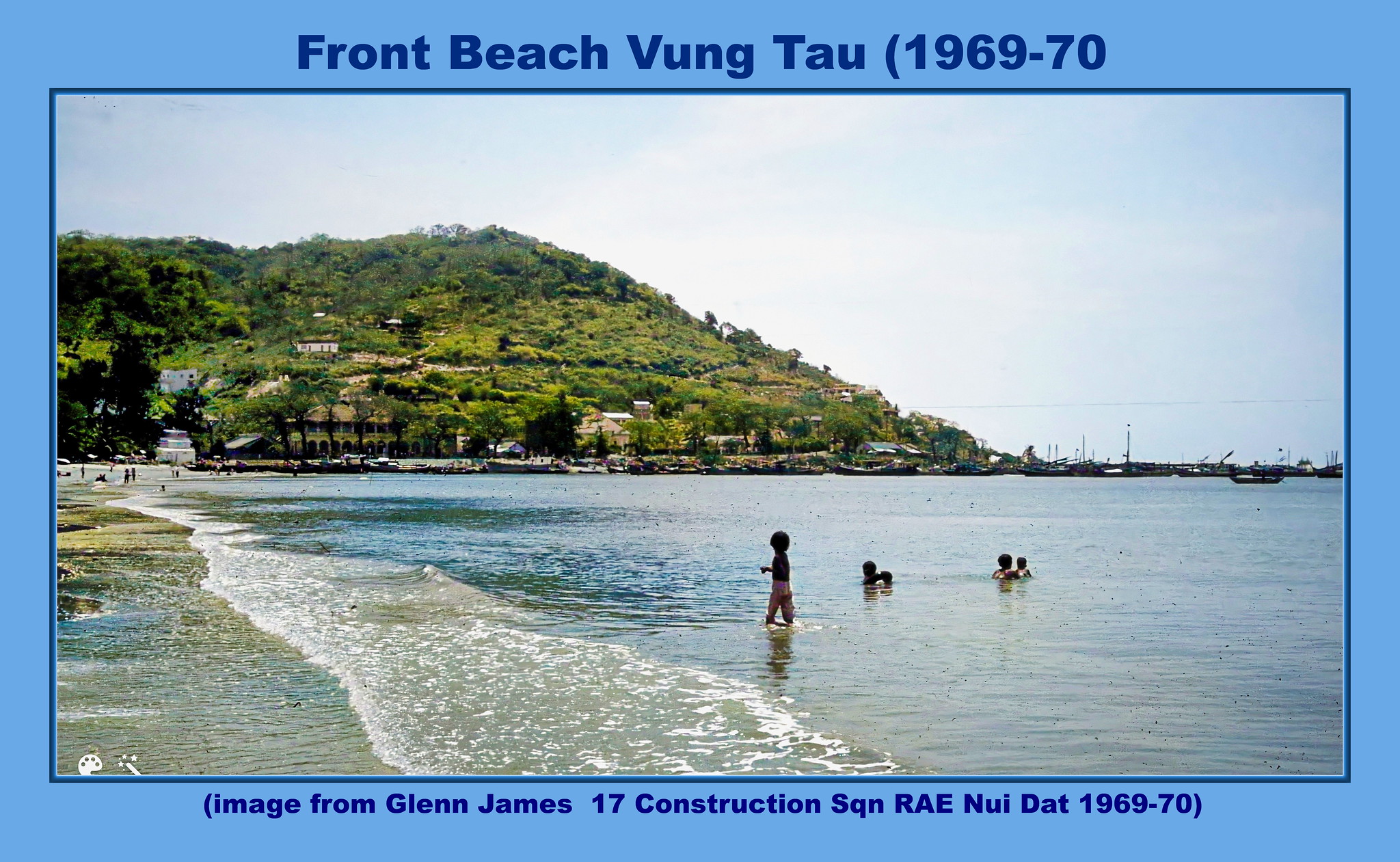This image, framed with a thick light blue border and dark blue text, captures a serene beach scene labeled "Front Beach, Vung Tau, 1969-70." Below the photograph, text credits the image to Glenn James, 17 Construction Squadron, RAE, Nui Dat, 1969-70. The photograph showcases a beautiful beach where a few children play in shallow bluish-gray water with light waves gently lapping at the shore. In the distance, multiple boats are docked against a backdrop of a lush, green hill adorned with trees, shrubbery, and scattered buildings. Above, a light blue sky is dotted with bright white, opaque clouds. The beach itself is sparsely populated, with a sandy shore visible on one side and vibrant, multi-hued water on the other.